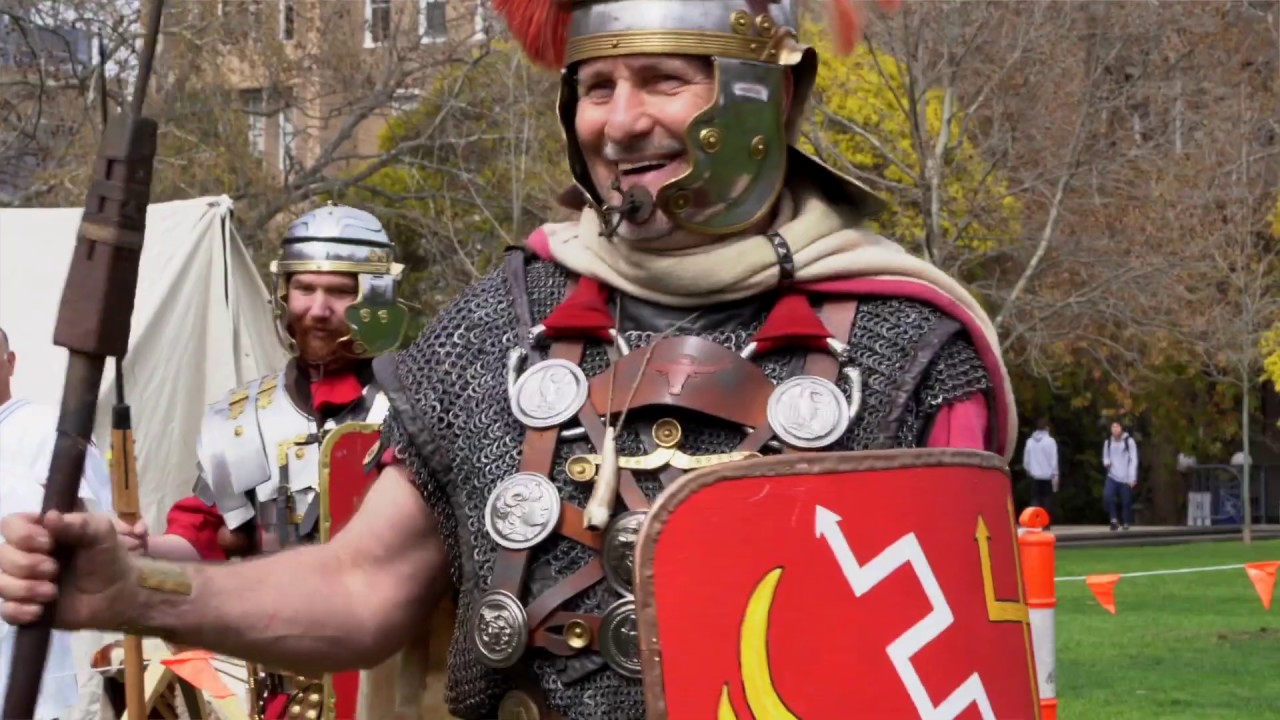In this detailed image, we see a vibrant scene reminiscent of a medieval festival, possibly taking place in a well-manicured park, likely on a college campus. The central figure in the foreground is strikingly dressed as a Roman centurion, donning chain mail armor, a metal helmet, and a leather bracing across the chest. In his left hand, he firmly grasps a colorful red shield adorned with intricate white and yellow designs, while his right hand holds a pike-like spear. Accompanying him is another individual in period costume, slightly behind and to the right, who is similarly equipped with a silver helmet and chain mail. This person holds a spear with a wooden handle and a black tip. 

To the left of the main figures stands a canvas tent, evoking a sense of historical immersion. Further in the background stands another person, possibly a clergy member or historical figure, dressed in a simple white robe. The backdrop features a multi-story stone or brick building, adding an interesting juxtaposition between the historical reenactment and the modern environment. 

Also visible are modern elements such as caution tape with orange flags and two individuals in contemporary clothing—jeans, light-colored jackets, and a backpack—walking in the distance, enhancing the image's blend of past and present. A tree with vibrant yellow leaves or blooms contributes to the scenic elegance of the setting, completing this richly detailed and dynamic tableau.